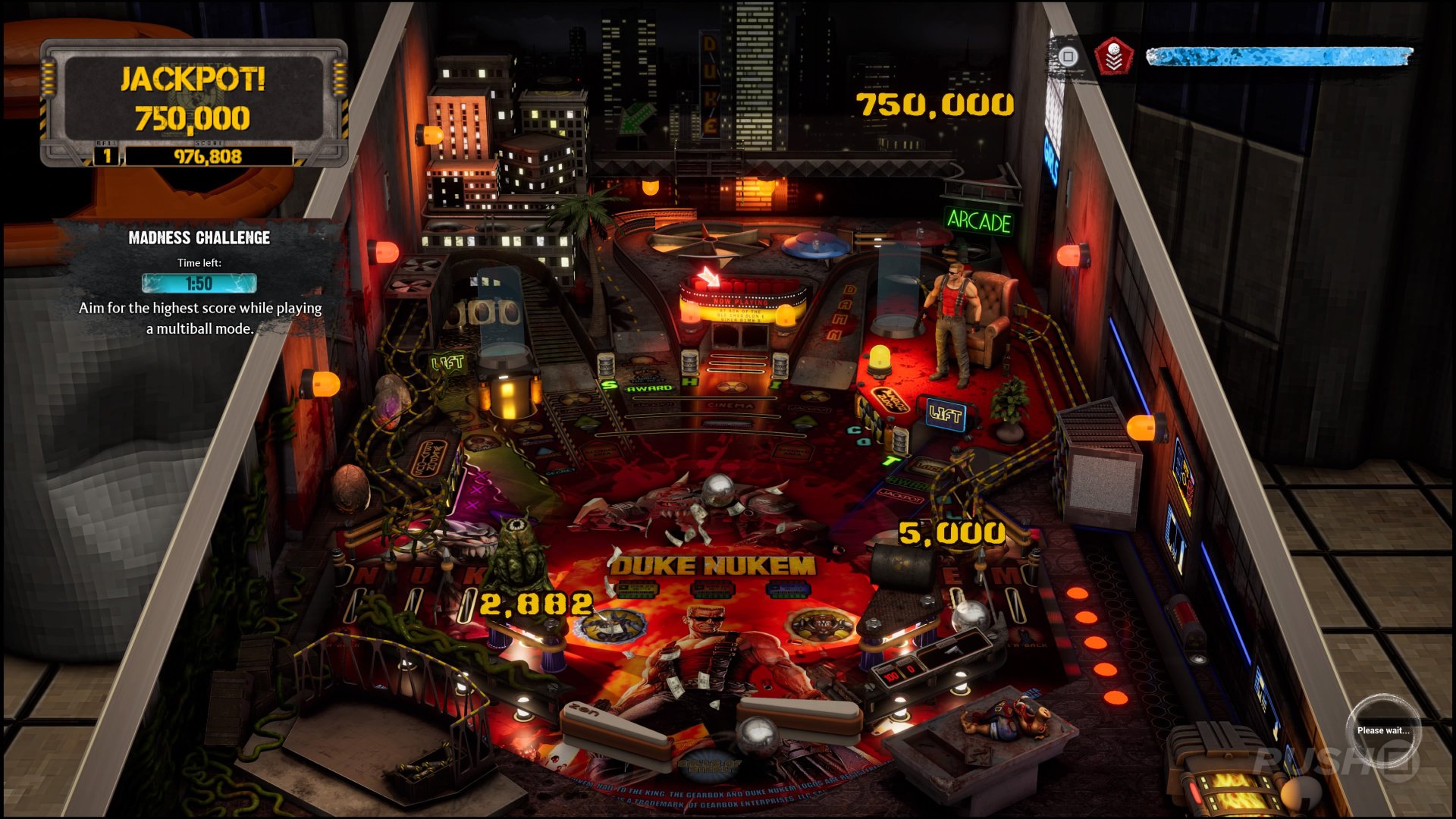The close-up image showcases a detailed representation of a Duke Nukem-themed pinball machine, likely a digital recreation rather than a physical pinball machine, due to the presence of floating heads-up displays and indicators. Dominating the scene is the muscular character Duke Nukem, depicted wearing a red tank top, black pants, and a bandolier of machine gun ammunition, with his figurine featured prominently in the top right corner. Below this, the machine's design incorporates paddles or flippers at the bottom, with a ball poised behind one, suggesting a game over scenario. The machine displays various scores: 2,882 in yellow on the left, 5,000 on the right, and a staggering 750,000 at the top right, while the current score clocked in at an impressive 976,808. Other annotations include "Jackpot $750,000" and "Madness Challenge" with a time indication of "1:50" in the top left, encouraging players to aim for the highest score in multi-ball mode.